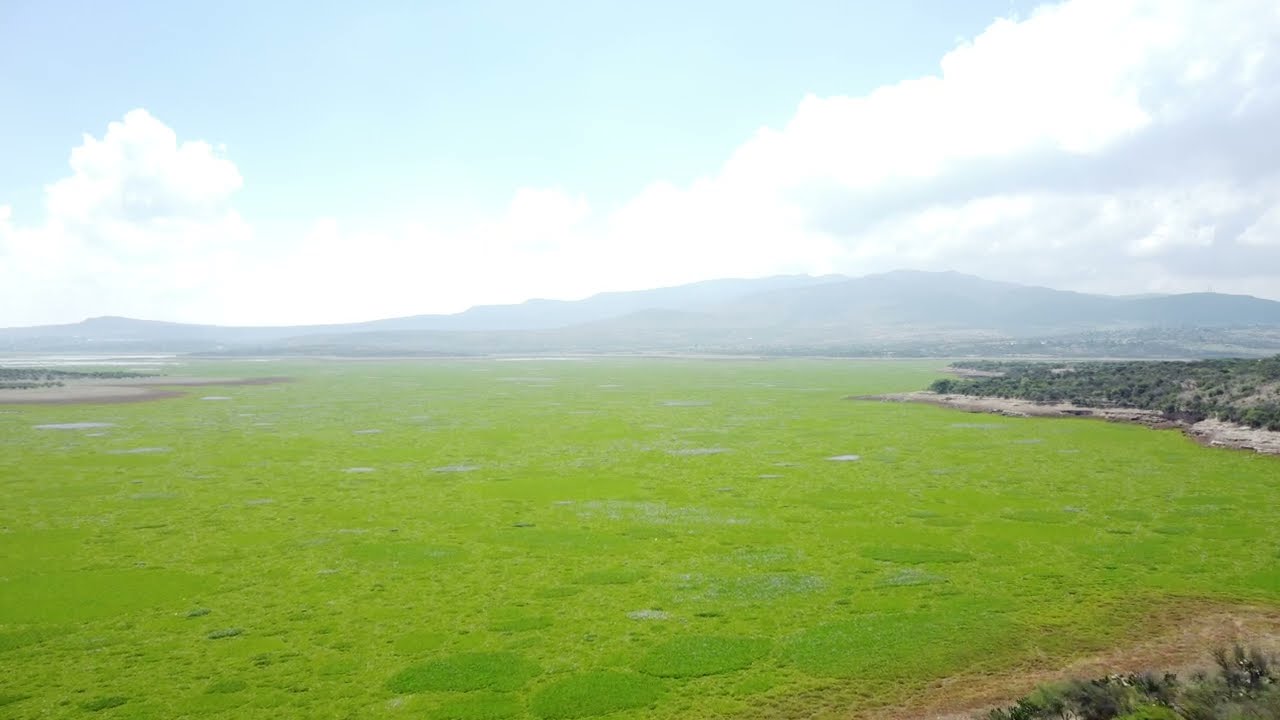The image is a high-angle shot, possibly taken from a hill or by a drone, capturing an expansive, lush, green valley extending for miles. The valley is predominantly covered in tall grasses, creating a near-seamless sea of green, with occasional blue patches suggesting water puddles within the grass. To the left, sandy dirt areas and what appears to be a serpentine river, winding down toward a large lake, add to the landscape's diversity. In the foreground, small shrub-like vegetation dots the area, while the dry, greener edges give way to a dry landscape with minimal vegetation. On the right, hills adorned with smaller trees rise up, leading the eye to larger, hazy mountains in the background. The mountains descend into a bowl shape where the grass starts growing, and the scene is framed by a mix of clouds and clear skies, providing a serene yet dynamic backdrop. In the top right of the image, a low cloud line forms just behind the mountains, adding depth and texture to the picturesque scene.